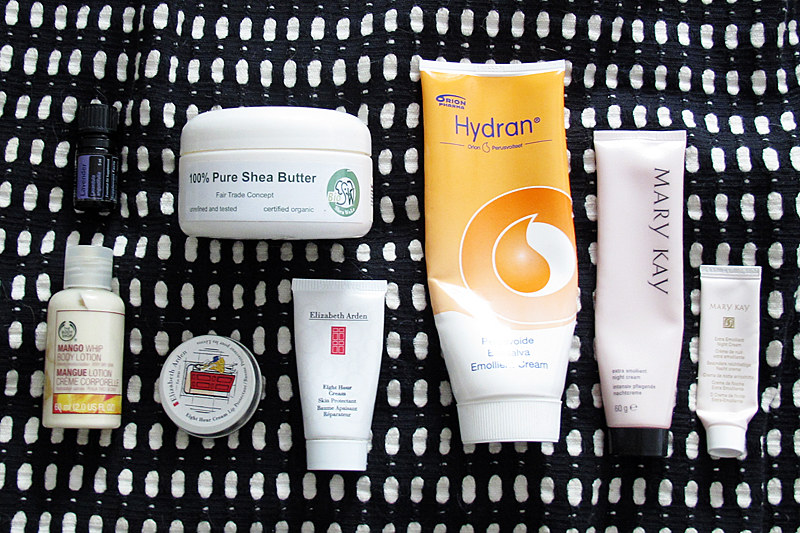The landscape-oriented photograph showcases a selection of skincare products meticulously arranged on a black cloth adorned with white vertical, jelly bean-like shapes and small white dots interspersed between them. These intricate patterns are sewn into the fabric, emphasizing craftsmanship. 

The composition features eight products, aligned from right to left:

1. **Mary Kay Squeeze Bottle**: This small, light pink tube resembles a travel-size, flattened toothpaste tube. It has a white, flat cap at the bottom and displays the brand name "Mary Kay" at the top, followed by a square logo and about ten lines of diminutive lettering in light brown.

2. **Mary Kay Large Bottle**: A taller, wider counterpart to the first, this bottle is primarily pink, with "Mary Kay" written in black and oriented 270 degrees along the right side. The cap is black, situated at the bottom, above which are four lines of small black text indicating its capacity of 50 grams.

3. **Hydrant Sun Cream**: An even larger, orange bottle with a white cap at the bottom. The text "Hydrant" and the logo "Orion" are printed in blue near the top. The lower right features a darker orange circle with an orange raindrop design. A white band near the cap contains blue text that is partially obscured by light reflections, likely stating "emollient cream."

4. **Elizabeth Arden Mini Bottle**: Positioned to the right, this small white bottle with a white cap carries the brand name "Elizabeth Arden" at the top. It features a red rectangle and tiny black text near the bottom, indicative of a travel-sized cream.

5. **100% Pure Shea Butter Container**: A white plastic jar with a white label, displaying dark green text that reads "100% Shea Butter." It includes a circular green logo on the right side of the label.

6. **Elizabeth Arden Lip Balm**: A small metallic circular container marked with "Elizabeth Arden" around its edge. The center image is ambiguous but appears to be reddish.

7. **Mango Body Lotion**: A small, hard plastic bottle with a clear cap. The label is light pink with orange outlines, stating "Mango Whip" and "Body Lotion," with translations in different languages including "mankay lotion crème."

8. **Small Dark Bottle**: The final item is a tiny, nearly black or dark purple glass bottle with a black cap. Its design suggests it might be an extract bottle, though the exact content is not specified.

The detailed arrangement on the intricately patterned cloth highlights the diversity of the skincare products, along with their distinct branding and packaging.